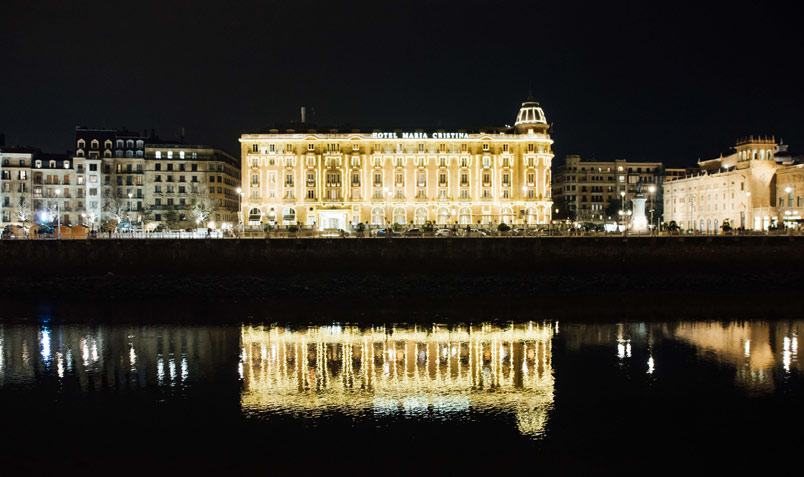A breathtaking nighttime cityscape captured from across a body of water, showcasing the beautifully illuminated Hotel Maria Cristina at the center. The hotel, a grand and regal four-story structure, stands adorned with warm yellow-golden lights that accentuate its old-world, European elegance. On the right side of the roof, a small, intricately lit dome with two concentric circles highlights the building’s architectural splendor. The surrounding buildings are mostly unlit, drawing focused attention to the hotel. In front of the hotel, a busy street can be seen with street lights and multiple cars. The reflective waters in the foreground mirror the lit buildings, adding a serene contrast to the dark, moonless night sky. The entire scene emanates a vintage, royal charm, making the Hotel Maria Cristina the undisputed centerpiece of this enchanting urban landscape.